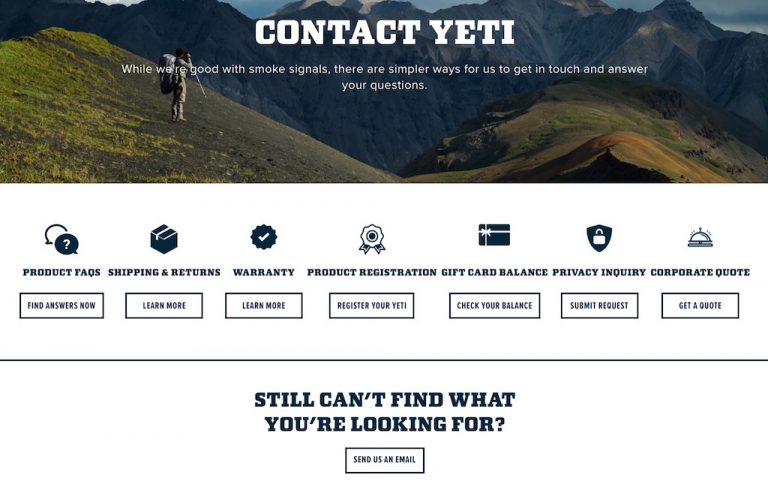In this captivating advertisement for a website, a breathtaking landscape of lush, rolling mountains unfurls across the image. Dominated by verdant greenery, the scene is serene and tranquil. Positioned on the upper left side of the image, a lone hiker equipped with a backpack and a walking stick appears to be embarking on an adventurous journey through this picturesque terrain. Overlaying this scenic backdrop, bold white text reads, "Contact Yeti."

The text continues, humorously noting, "While we're good with smoke signals, there are simpler ways for us to get in touch and answer your questions." Below this, various contact options are listed from left to right to assist users. The options read as follows:
- "Still can't find what you're looking for? Send us an email."
- Above this: "Product FAQs. Find answers now."
- To the right: "Shipping and Returns. Learn more."
- "Warranty. Learn more."
- "Product Registration. Register your Yeti."
- "Gift Card Balances. Check your balance."
- "Privacy Inquiry. Submit Request."
- "Corporate Quote." Accompanied by a charming illustration of a desk bell, this option reads, "Get a Quote."